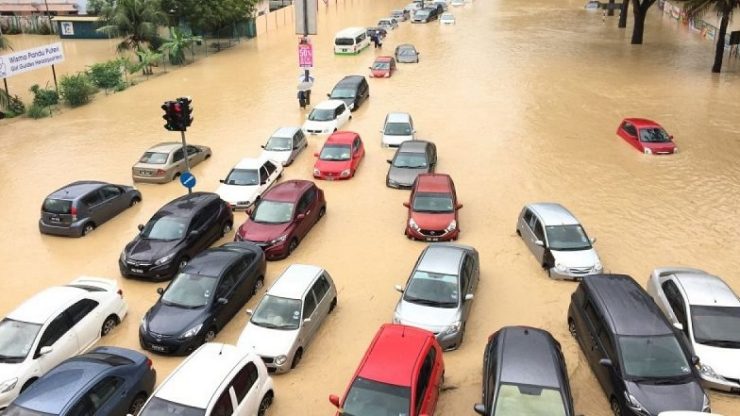This photograph, taken from an elevated vantage point in a flood-stricken town, vividly captures a road overwhelmed by muddy, light brown floodwaters. The inundated street is teeming with dozens of vehicles, including small sedans, hatchbacks, and compact SUVs, of various colors such as silver, red, black, and dark red. The cars in the foreground form multiple rows, with floodwaters reaching up to their wheels, while those in the background are almost halfway submerged. Amidst this chaotic scene, there are streetlights and signboards visible, with one notable white sign with blue text situated in the upper left corner. Surrounding this flooded thoroughfare are plants, lower green trees, and bushes, partially submerged by the floodwaters, along with a small wooden fence and a blue-green hut or building in the upper left. The trees in the upper right corner also have water partway up their trunks, further emphasizing the severity of the flood. This detailed shot not only highlights the extent of the flooding but also the various elements - both man-made and natural - that are immersed in the murky waters.